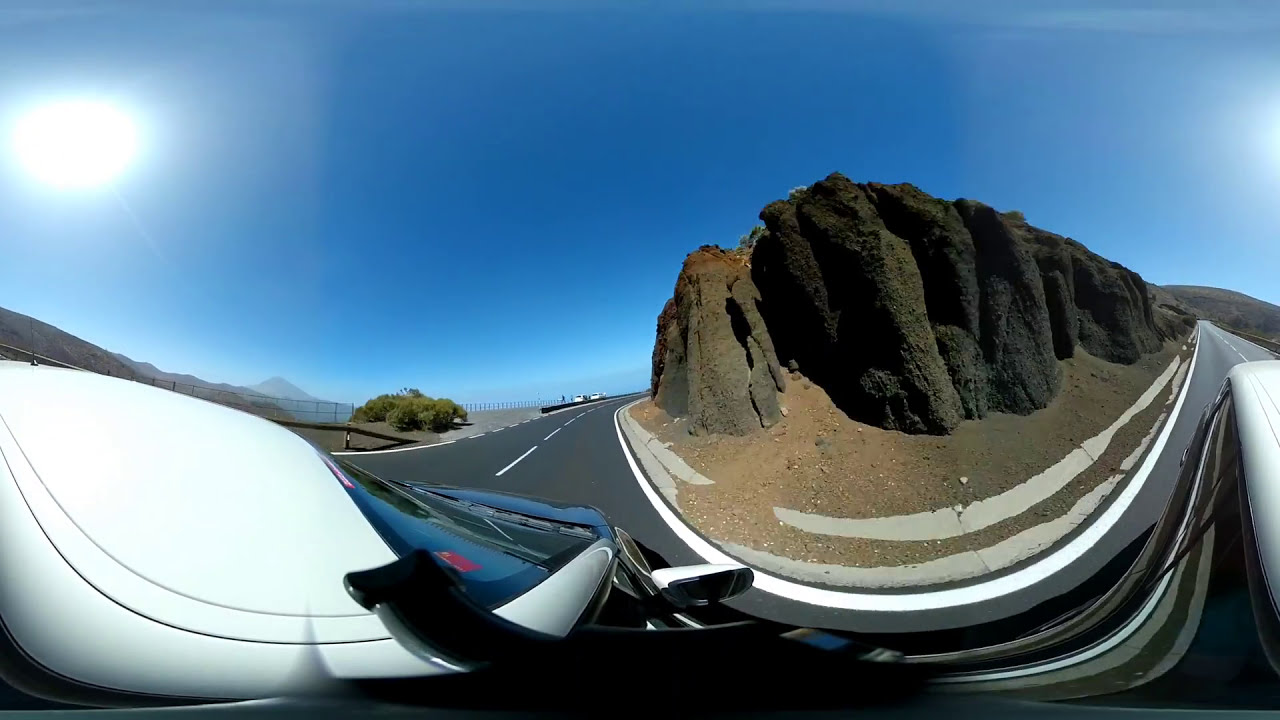A narrow and curvaceous highway loops around a central rock formation, creating a potentially dangerous and tight-turning road. The road, made of dark gray asphalt, is lined with white painted lines on the edges and in the center. The central rock formation, surrounded by a light brown concrete curb, starts with a light brown dirt base and transitions to gray rocks that become darker and greener towards the top. To the left side, part of a light-colored vehicle, including the windshield, is visible. The sky above is a gradient of light blue becoming darker towards the center, with a bright white light in the upper right corner and another on the far right edge. The scene is bathed in sunlight, contributing to a summertime vibe, with no clouds in sight. Surrounding the highway, there is green shrubbery and distant mountains, enhancing the naturesque appeal reminiscent of regions like New Mexico or Arizona. The curb's tightness and the road's curves contribute to its reputation as one of the most dangerous roads, adding to the caution required for drivers navigating through this scenic yet treacherous route.